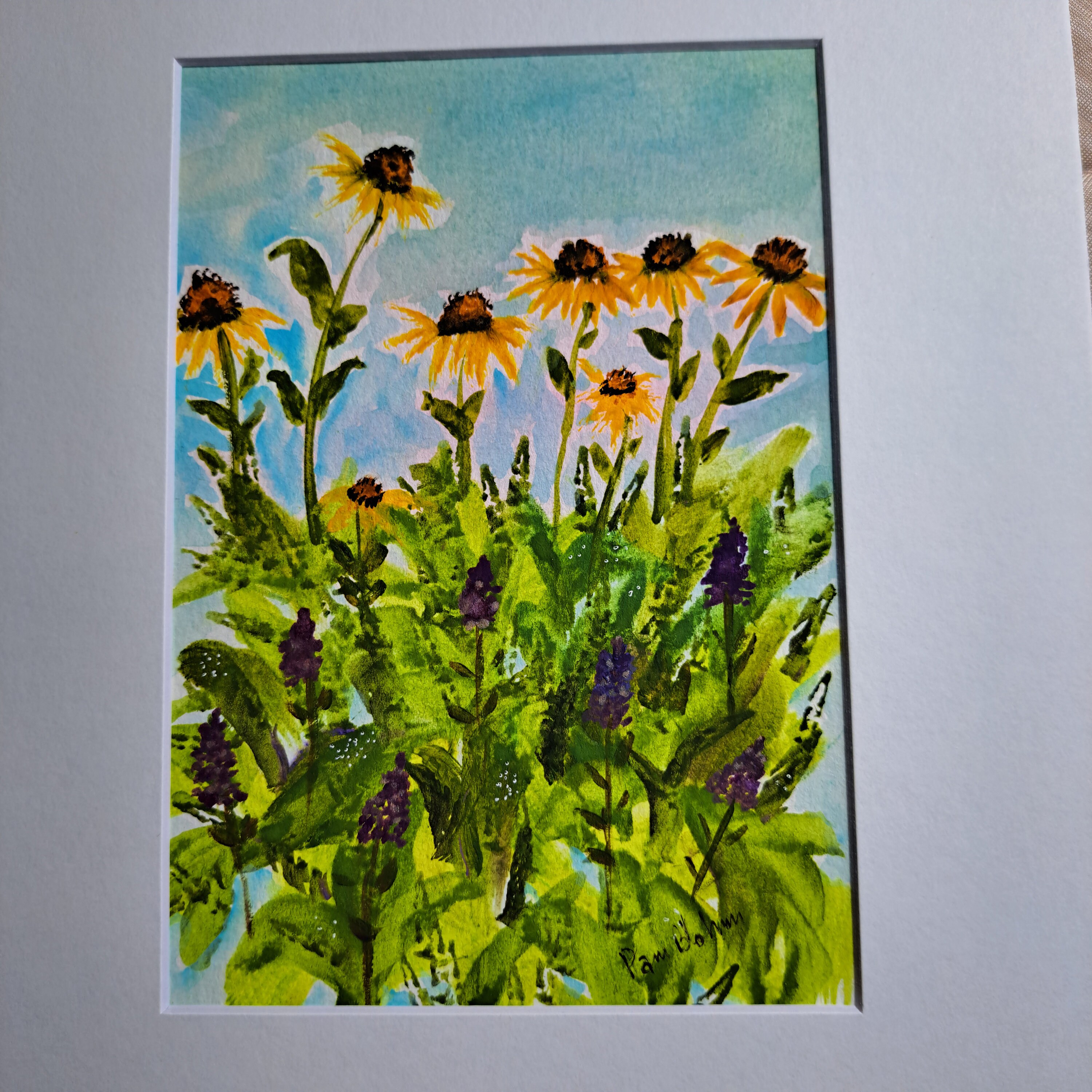The image depicts a vibrant watercolor painting framed in a large light blue, rectangular frame standing vertically. The focus of the painting is a group of bright yellow sunflowers, with six large ones dominating the top portion. Among these, the tallest sunflower leans slightly to the right. The left sunflower stands at an average height, and the third one is the shortest. The next three are of similar height but face different directions; the left one faces upward, the second slightly to the left, and the third to the right. Surrounding these sunflowers are delicate white wisps of clouds against a blue sky. Below the sunflowers are additional flower buds that have not bloomed yet, appearing as almost-black bulbs amidst long green leaves. At the bottom of the painting, a distinct arrangement of purple flowers, likely made up of tiny purple balls giving them a triangular shape, contrasts with the yellow sunflowers above. The entire scene is signed at the bottom by an artist named Pam, though the last name is unclear.